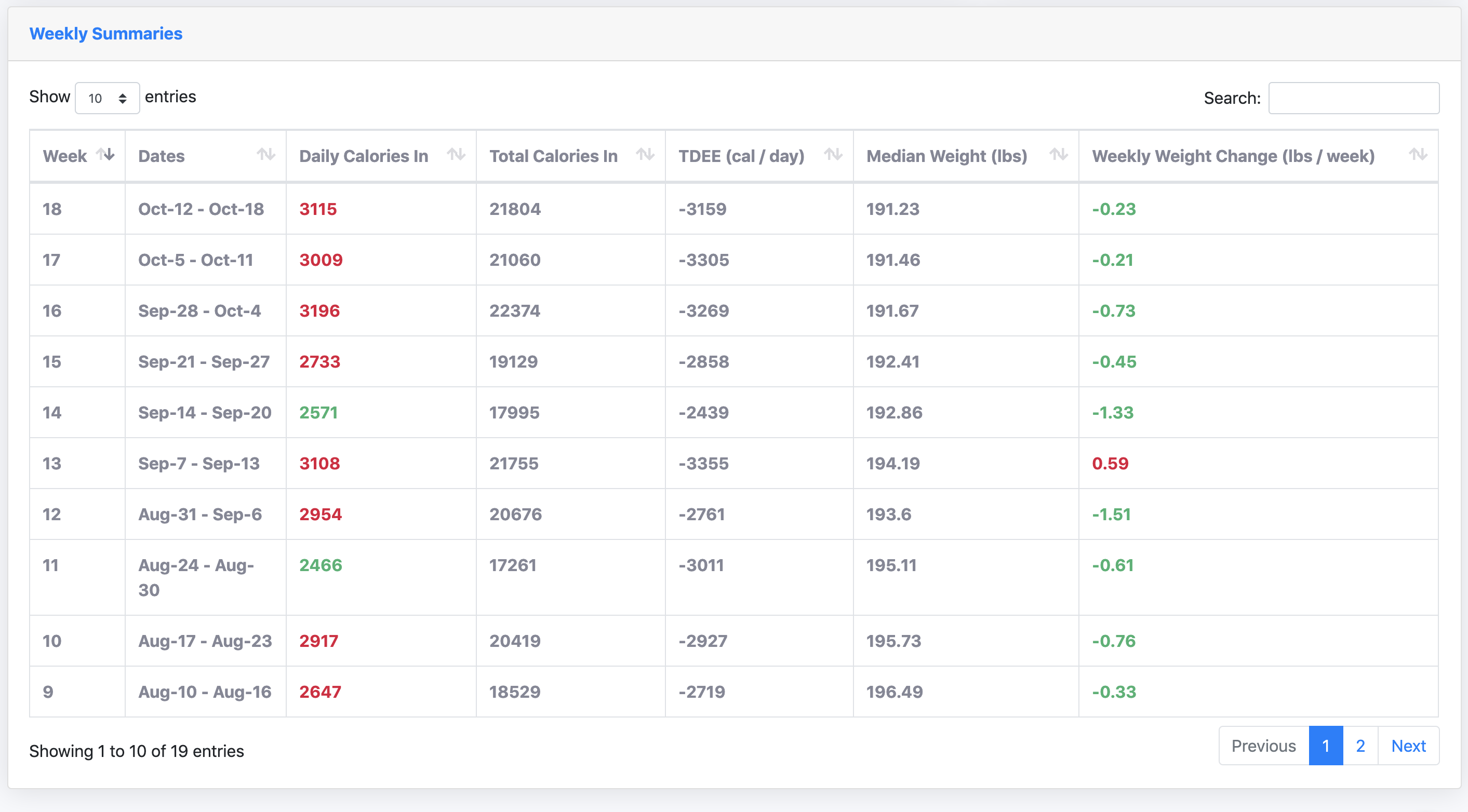The image depicts a detailed horizontal chart against a white background, titled "Weekly Summaries" in blue font at the top left corner. Below the title are a scroll bar indicating the number of entries and a search box located at the far right. The chart is organized into seven categories, each labeled in bold gray font, encompassing the following columns: Week, Dates, Daily Calories In, Total Calories In, TDEE (Total Daily Energy Expenditure), Calories Per Day, Medium Weight in Pounds, and Weekly Weight Change in Pounds per Week. 

The chart lists weeks in descending order, from Week 18 to Week 9. At the bottom left corner, black text indicates "Showing 1 to 10 of 19 entries." Meanwhile, the bottom right corner features the current page number, with "1" being selected, denoting it as Page 1. Adjacent to this are the number "2" and the word "Next" for navigation. 

The "Weekly Weight Change" column uses green or red font to highlight whether the person experienced weight loss or gain, respectively. Similarly, the "Daily Calories In" entries are color-coded, with red and green fonts indicating different values.